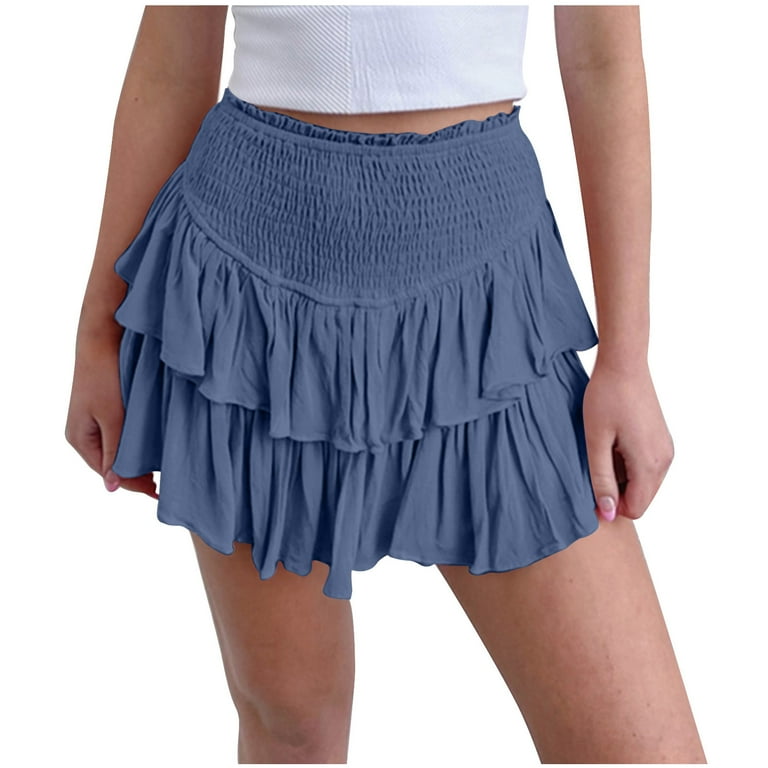The image depicts a Caucasian woman standing against a plain white background, visible from just below her chest to her knees. She wears a white knit top that exposes a small strip of her midriff. Her lavender, periwinkle, or bluish-gray skirt, made from a cotton-polyester blend, is very short, ending at her mid-thighs. The skirt features an elastic waistband that extends from her hips up to her belly button, with a ruffled, two-tiered design. The woman stands with her weight shifted onto her right leg, her left leg slightly extended, and her arms resting at her sides with her fingers curled under and thumbs pointing down. Additionally, she sports pink nail polish on the tips of her fingernails.